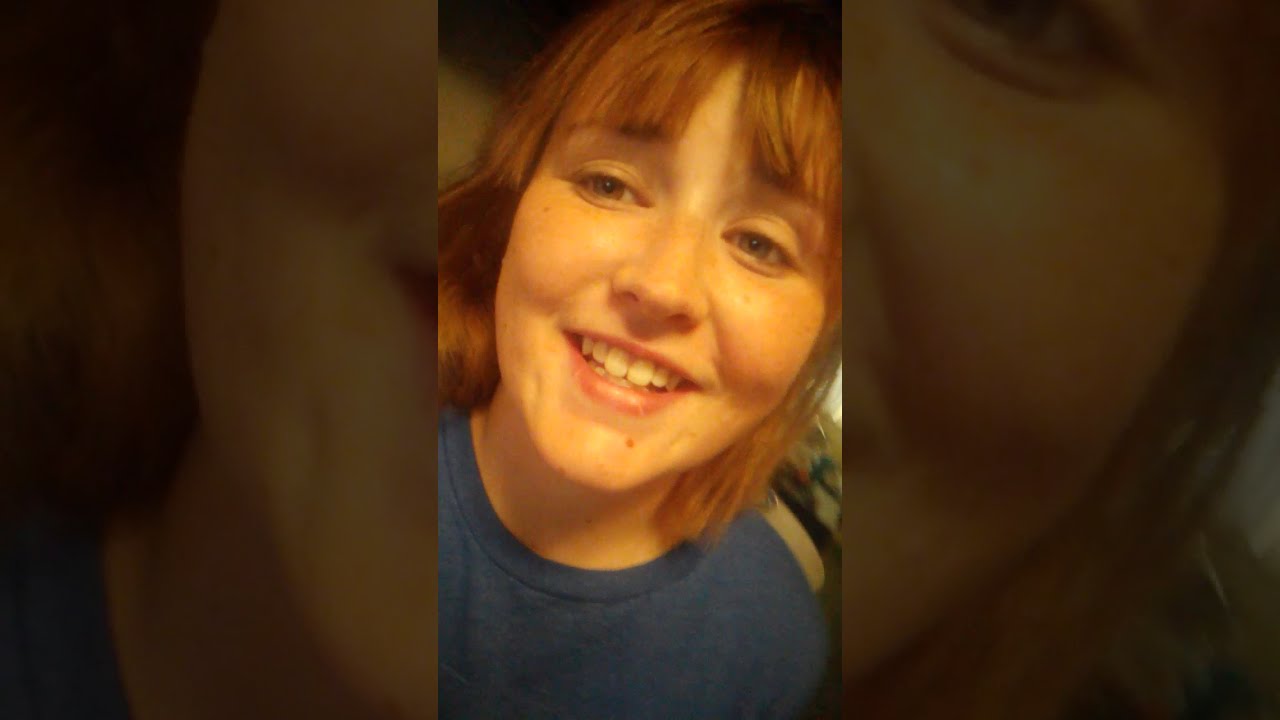The image features a smiling young woman with short, shoulder-length brown hair that has a hint of red and is styled with bangs forming a slight V-shape at her forehead. She has light-colored eyes that sparkle in the warm, golden lighting, enhancing the friendly and inviting atmosphere. The woman is dressed in a dark blue t-shirt, visible from her torso upwards.

The photograph is a vertical selfie, common to smartphones, but uniquely arranged into a horizontal rectangle divided into three smaller panels. The left and right panels are close-up, darker, and highlight the right and left sides of her face, respectively. The central panel, which is slightly smaller and superimposed over a muted background version of the same photo, shows her entire face more clearly and brightly, with her head slightly tilted to the right. Her open smile reveals her teeth, and a portion of her hair at the top edges of the middle panel is cropped out. This artistic arrangement gives the image a dynamic, almost video-reel-like feel, reminiscent of social media formats like YouTube Shorts or TikTok.